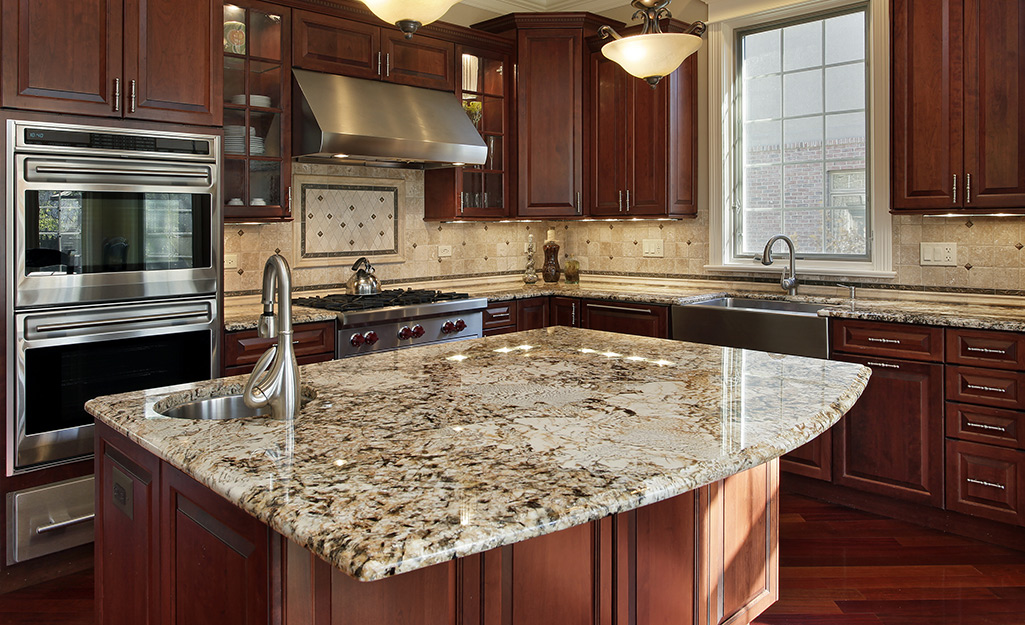This detailed photograph captures an elegant kitchen that features a rectangular layout, wider than it is tall, with an array of both modern and traditional elements. The kitchen is dominated by rich, dark-stained mahogany cabinetry, complemented by a lighter brown travertine backsplash adorned with darker accents. At the center of the kitchen is a freestanding island with a rounded, light brown marbled countertop, which also houses a silver sink and faucet on the left-hand side. 

The stainless steel appliances add a modern touch, including a large gas range with a hood vent and a double wall oven on the left, distinguished by their sleek silver finish and red detailing on the range's knobs. The floor, in a slightly lighter shade of brown than the cabinetry, exhibits a warm wood texture, harmonizing the overall earthy palette of the room.

On the right-hand side, a large window with silver bars set in square-shaped patterns allows natural light to flood the space, enhancing the kitchen's inviting atmosphere. The window is situated above additional cabinetry and a sink area. Two pendant ceiling lights with rounded bulbs hang down, providing additional illumination to the central island area.

Additional details include the silver hardware on the cabinet doors and drawers, a silver kettle on the stove, and a few glass-fronted cabinets that display dishes, adding both functionality and aesthetic appeal to this meticulously designed kitchen.